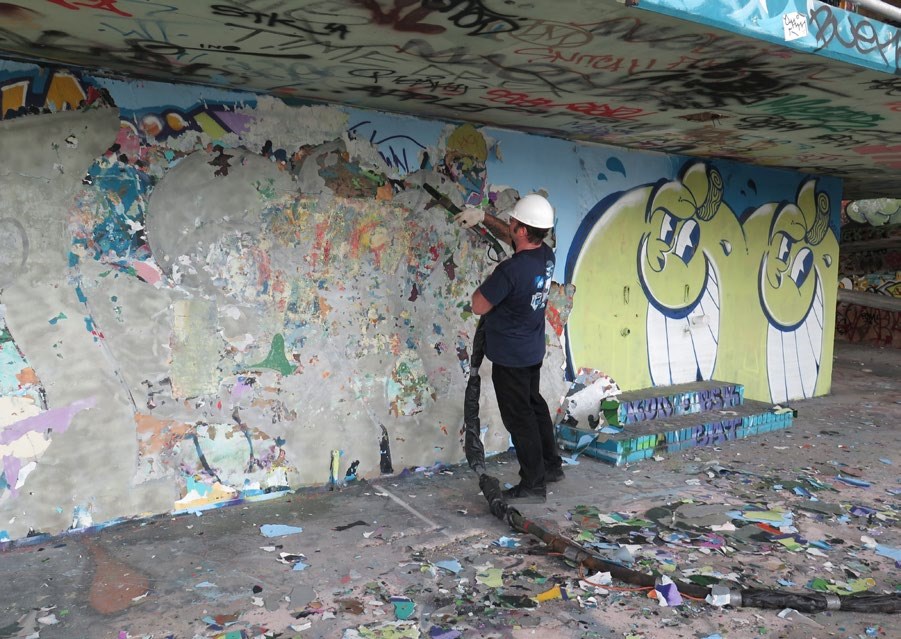In this outdoor scene, a man wearing a white construction hard hat, a navy blue shirt, black jeans, and black shoes is diligently working to remove graffiti from a concrete wall. He sports short black hair and probably a beard and is wearing rubber gloves for protection. Equipped with a tool that seems to be either a power sander, high-pressure hose, or sand blaster—wrapped with duct tape—he is actively chipping away at the graffiti, leaving a trail of chipped paint at his feet. The wall he is working on is part of a structure that includes a concrete slab floor and a roof above, both heavily adorned with colorful graffiti in various styles and words. To the right side of the wall, two pieces of graffiti depict green apples with cartoonish faces showing their teeth, still intact amidst the ongoing cleanup. The setting appears to be under a bridge, where different kinds of graffiti and some sort of plaster have created a chaotic visual palate, which the man is methodically clearing away.